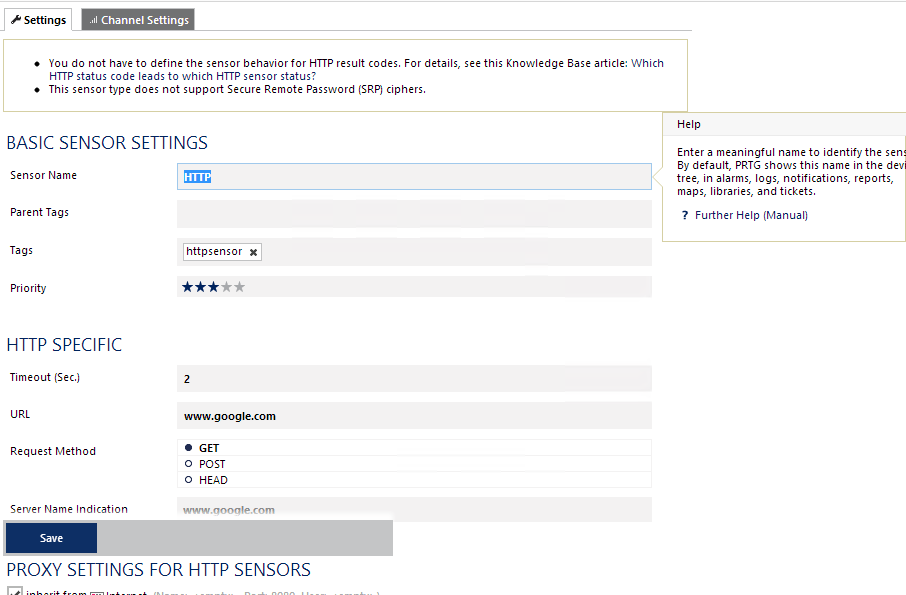This photo captures the detailed view of a channel settings tab within a web interface. At the top left, there's a "Settings" tab accompanied by a small wrench icon. Adjacent to the right, a "Channel Settings" tab is highlighted in gray, indicating it is the currently active section.

Below these tabs, there's a prominent information box. The first bullet point within the box reads, "You do not have to define the sensor behavior for HTTP result codes. For details, see this knowledge base article which HTTP status code leads to which HTTP sensor status," with a blue, hyperlinked text directing users to the article. The second bullet point states, "This sensor type does not support Secure Remote Passwords (SRP) ciphers."

Further down the web page, under the main body, the section titled "Basic Sensor Settings" is visible, containing various options. There's a field labeled "Sensor Name," which has an input box next to it. The text "HTTP" is entered in this box, highlighted in light blue. To the right of this input box, a help pop-up description reads, "Help: Enter a meaningful name to identify the sensor. By default, PRTG shows this name in the device tree, alarms, logs, notifications, reports, maps, libraries, and tickets." At the bottom of this section, a question mark icon linked to "Further Help Manual" is also hyperlinked in blue.

The image effectively showcases the comprehensive functionalities and settings available for configuring a sensor within the interface.